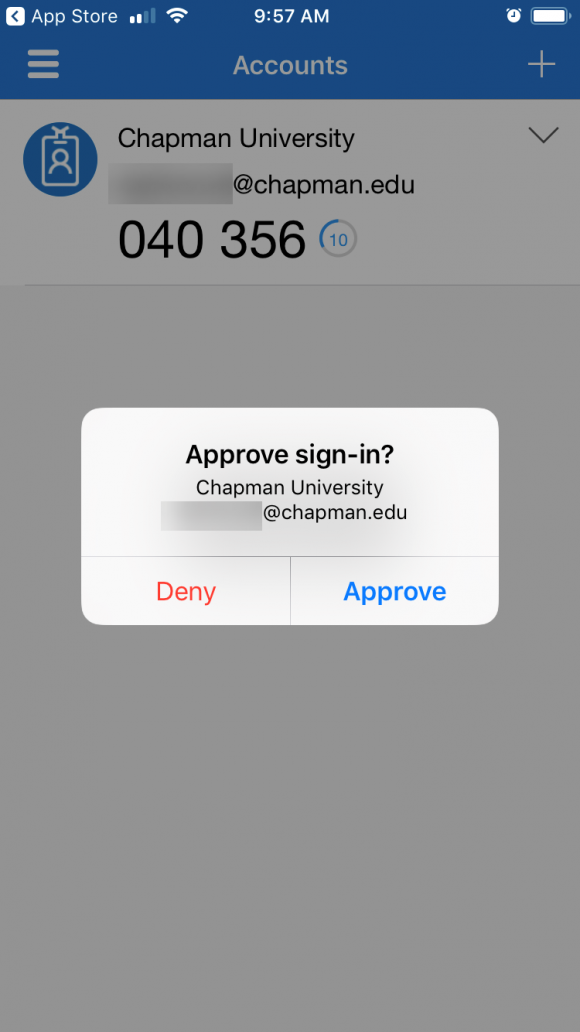The top portion of the image is a blue header resembling a screenshot from a smartphone. At the top left of the header, the text "App Store" is displayed in white. The status bar shows a strong Wi-Fi signal with all bars filled in white and the time reads "9:57 a.m." next to a clock symbol and a fully charged battery icon, both in white. 

Below this header, the screen transitions to a gray background where the visual content is obscured by a pop-up notification. Before the pop-up appeared, the screen displayed text reading "Chapman University" in black, with a partially obscured email address "appchapman.edu" in black, and the sequence "040356". 

The pop-up notification is rectangular and light gray. At the top, in black text, it says "Approved" with a capital 'A', followed by "Sign-In?" Below this line, it again lists "Chapman University" with the same partially visible email address "appchapman.edu". There is a thin horizontal line separating the sections of the pop-up. 

At the bottom of the pop-up are two buttons: the first is a red button labeled "Deny" in white text, and the second is a blue button labeled "Approve" with a capital 'A' also in white text.